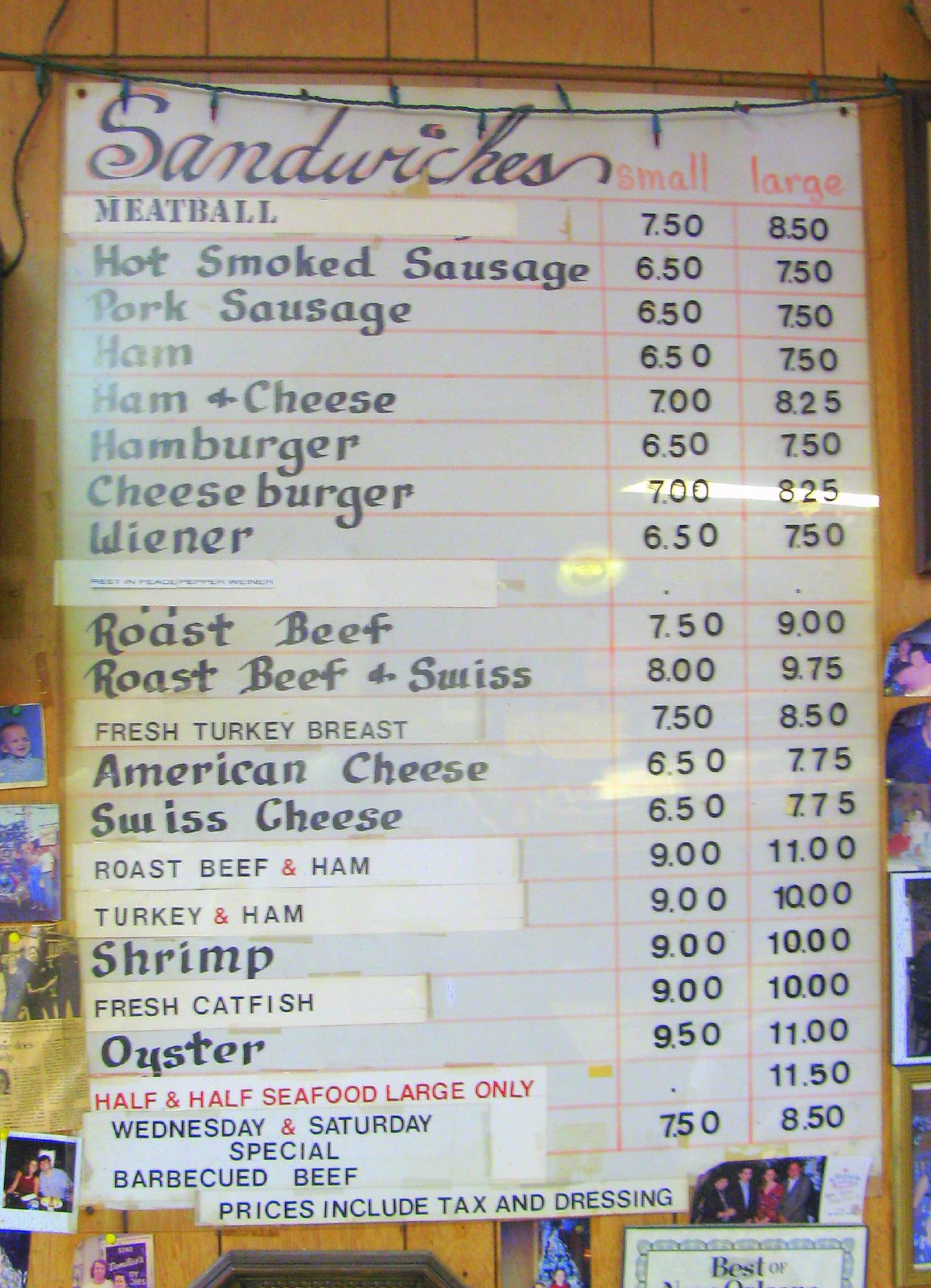This photograph features a rustic sandwich board, typical of a roadside restaurant, prominently displayed against a paneled wall. The board, adorned with Christmas lights at the top, proudly announces "Sandwiches" in black cursive writing over a pink background. Below this heading, the board details various sandwich options and their corresponding prices for small and large sizes.

On the left-hand side of the board, a diverse array of sandwich choices is listed, including meatball, hot smoked sausage, pork sausage, ham, ham and cheese, hamburger, cheeseburger, wiener, roast beef, roast beef and Swiss, fresh turkey breast, American cheese, Swiss cheese, roast beef and ham, turkey and ham, shrimp, fresh catfish, oyster, half and half, and seafood (available in large only). Additionally, it mentions a special barbecued beef sandwich available on Wednesdays and Saturdays. All prices include tax and dressing.

The sign is flanked by personal touches, such as family photographs, including a Polaroid picture of a young child and a "Best of" award, adding a warm, community-oriented feel to the restaurant's ambiance.